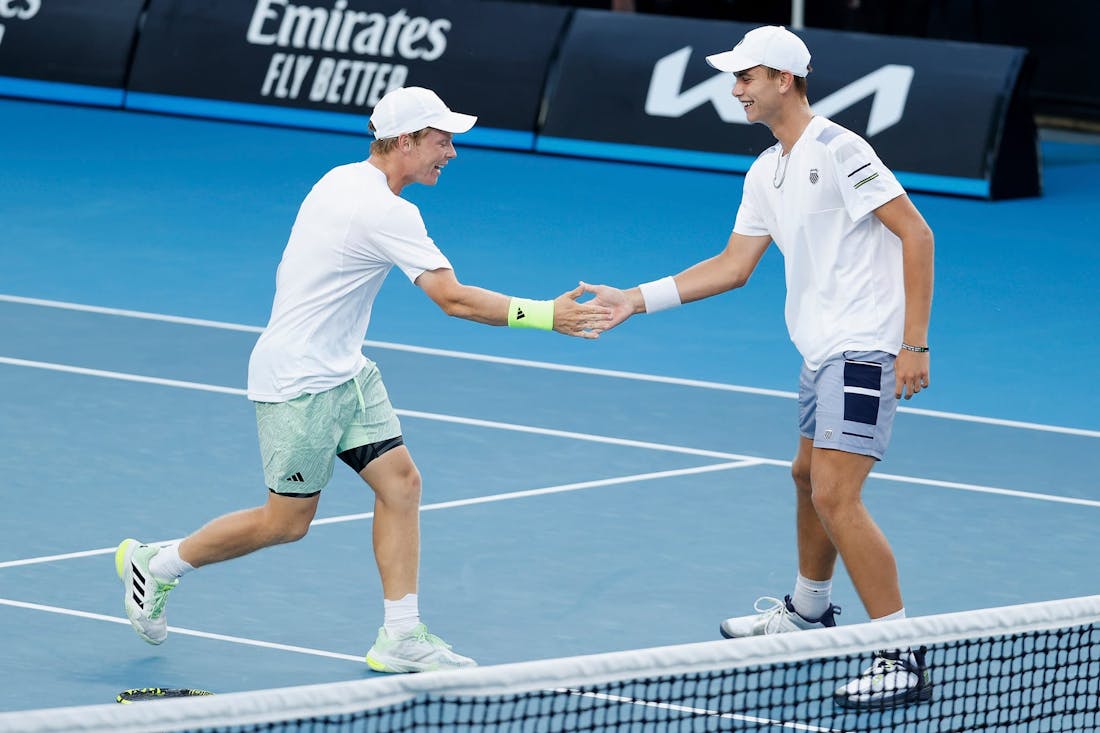Against the backdrop of an outdoor tennis court, two young men, seemingly in their 20s, are captured in a moment of camaraderie at the end of a match. The court itself is a vibrant light blue with white outlines, surrounded by a deeper royal blue perimeter. Visible at the bottom of the image is a tennis net, reinforcing the post-match scenario. Both players, each wearing white t-shirts and white baseball caps, are about to shake hands, smiling brightly. The left player, who appears Caucasian or European, sports mint green shorts and Reebok shoes, while the player on the right, who is possibly Arab or Latino, is slightly taller and dressed in darker, possibly gray-toned shorts. They each wear wristbands or wrist guards, enhancing the athletic vibe. Surrounding the court are dark blue sponsor barriers with signs promoting Kia and Emirates, adding a professional touch to the scene.